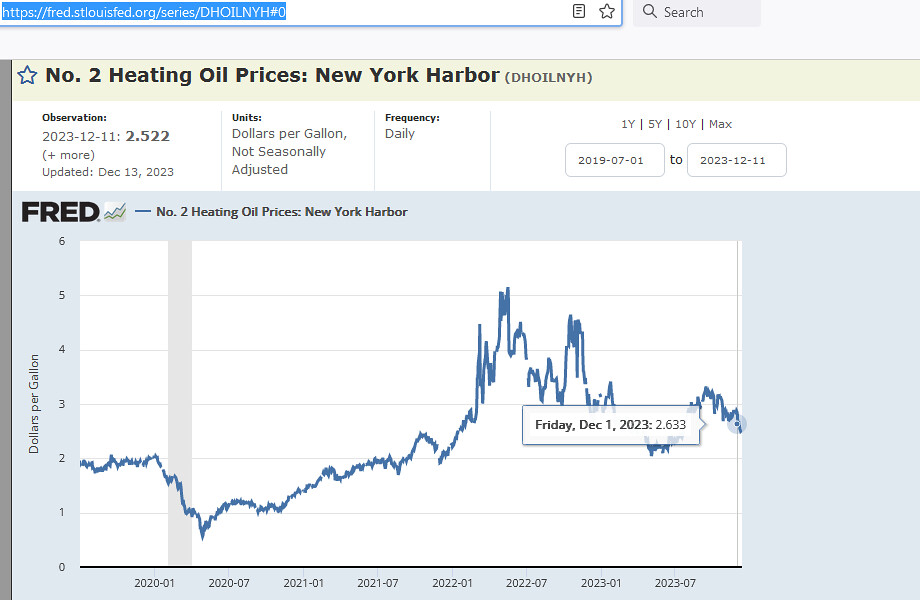The image is a detailed screenshot from a web browser displaying a line graph on a webpage. At the top, the browser's address bar shows the highlighted URL, "https://fred.stlouisfed.org/series/DHOILNYH," with a search bar to the right. The main content of the page features a heading and black text stating, "No. 2 Heating Oil Prices New York Harbor (DHOILNYH)," in a green banner. 

Beneath this, there are three information boxes:
1. The first box shows the observation date "2023-12-11" and a bold figure "2.522," updated on "December 13, 2023."
2. The second box lists units as "Dollars per Gallon, Not Seasonally Adjusted," in bold.
3. The third box states the frequency "Daily."

To the right, a date range menu offers options like "1Y, 5Y, 10Y, Max," displaying dates from "2019-07-01" to "2023-12-11."

The line graph itself features a blue line chart titled "No. 2 Heating Oil Prices New York Harbor," with a white background. The y-axis, labeled "Dollars per Gallon," ranges from 0 to 6, while the x-axis shows increments from "2020-01," "2020-07," "2021-01," "2021-07," "2022-01," "2022-07," "2023-01," to "2023-07."

The graph indicates a trend starting near the 2-dollar mark, dipping below 1 dollar, peaking at 5 dollars around 2022, and then gradually declining. A blue dot on the graph highlights "Friday, December 1, 2023," with a value of "2.633." The graph is surrounded by black and blue text, with finer details of dates and prices displayed prominently.